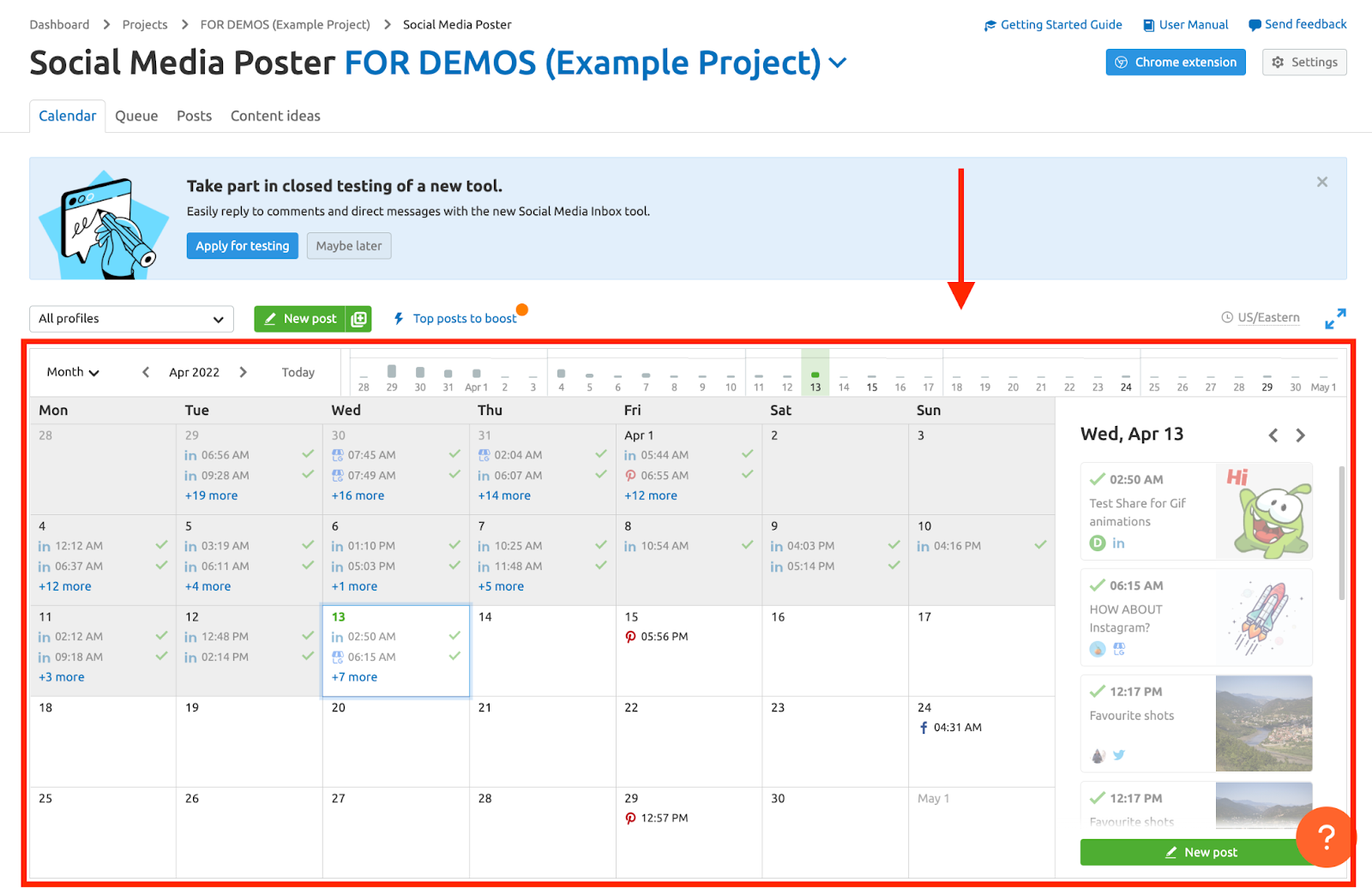This image is a detailed organizational layout for a social media campaign titled the "Dean Wolf Project." Dominating the visual is a large, red-bordered calendar for April 2022. The calendar spans from March 29th to April 30th, meticulously outlining scheduled posts across various social media platforms.

At the top of the image, there's a heading showcasing the origin of this project on a dashboard, specifically titled "Projects for Dean Wolf Social Media Poster." Below this, a secondary header reiterates the project's focus: "Social Media Poster for Dean Wolf." Adjacent to these headers, key components such as 'calendar,' 'cues,' 'posts,' and 'content ideas' are highlighted, indicating a structured approach toward planning.

A light blue information box stands out on the page, inviting users to participate in a closed testing phase for a new social media inbox tool, encouraging interaction through replies to comments and direct messages.

Delving into the calendar specifics, each date is filled with time slots for planned posts, characterized by a small icon representing the designated social media platform. For example, on April 7th, posts are scheduled for LinkedIn at 10:25 AM and again at 11:48 AM. Early entries, like April 1st, show detailed timings such as 5:44 AM and 6:35 AM, with mentions of multiple posts scheduled throughout the day.

The calendar exhibits a dense schedule up to April 13th, followed by sporadic entries on later dates such as the 15th, 24th, and 29th. This structure implies a significant push for content in the earlier half of the month with strategic, intermittent postings thereafter. The far-right margin of the calendar includes additional highlights, presumably marking notable dates or reminders pertinent to the Dean Wolf project.

Overall, the image encapsulates a well-organized and strategic social media campaign plan, ensuring consistent and timely dissemination of content across various platforms.